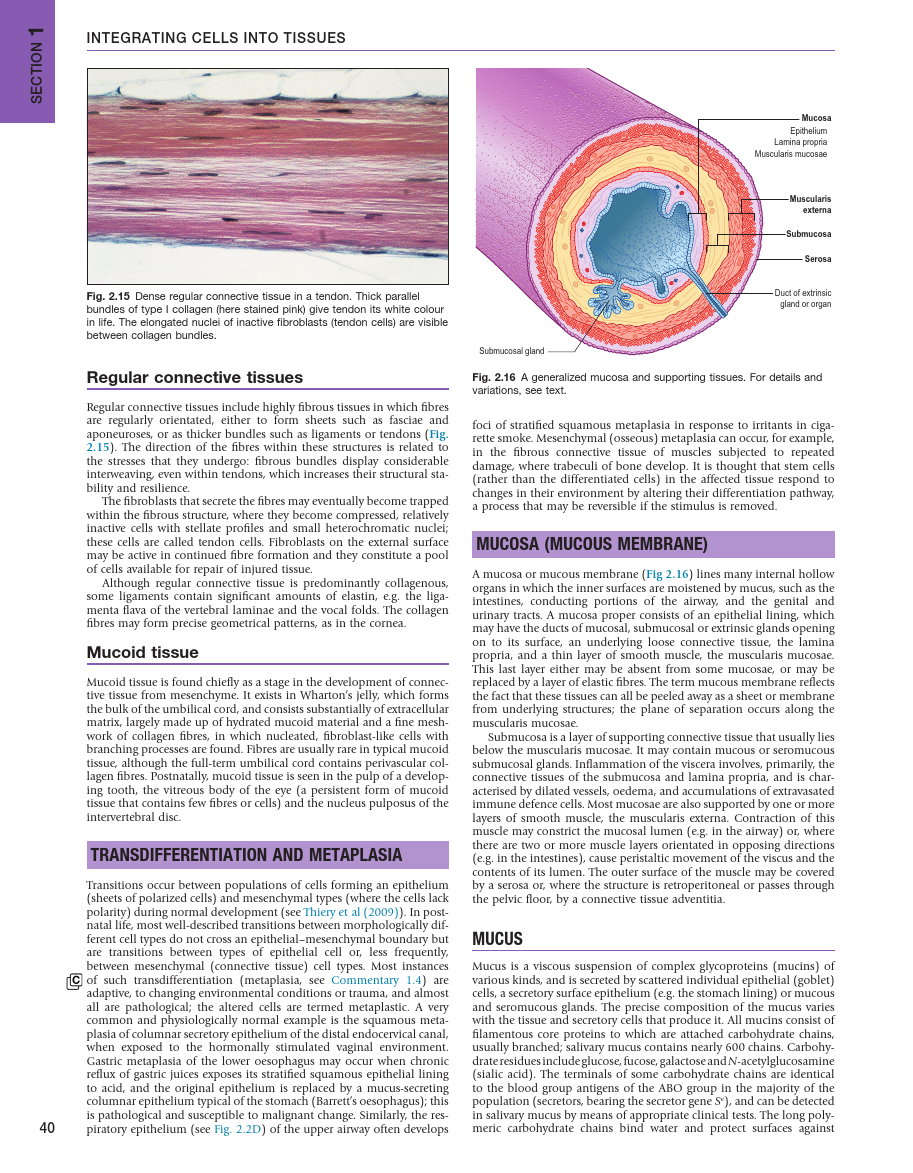This image is a detailed page from a biology textbook, marked as page 40 in the lower left corner. The top left corner features a vertical purple box labeled "Section 1," with the horizontal text "Integrating Cells into Tissues" beneath it. The page is formatted in two columns, typical of a textbook layout, and includes multiple sections and illustrations.

The first column begins with an illustration labeled "Figure 2.15: Dense Regular Connective Tissue." This diagram depicts thick parallel bundles of type I collagen, which are stained pink and showcased within a tendon. The text accompanying this figure explains that the elongated nuclei of active fibroblasts, also known as tendon cells, are visible between the collagen bundles. It describes regular connective tissues, where fibers are regularly oriented to form structures such as fascia, aponeurosis, ligaments, or tendons. These tissues help dissipate stress and provide structural stability and resilience. It mentions that active fibroblasts on the external surface of these tissues play a key role in fiber formation and repair.

Further down, the text discusses myxoid tissue, which is primarily found during the development of connective tissue from mesenchyme and is present in structures like the umbilical cord's Wharton's jelly.

In the right column, there is a description of transdifferentiation and metaplasia, with a specific mention of transitions between various cell types, often due to environmental changes or trauma. Examples given include gastric metaplasia in response to chronic gastric reflux and mesenchymal ossification in muscles subjected to repeated damage.

The second illustration, labeled "Figure 2.16: Generalized Mucosa and Supporting Tissues," provides a colored cross-section of tissue labeled with terms like mucosa, epithelium, lamina propria, muscularis mucosae, muscularis externa, submucosa, submucosal gland, and others. This figure helps explain the mucosa or mucous membrane, detailing its composition and functions across various internal organs. It also touches upon the structural attributes and roles of the different layers of the mucosa in health and disease.

Beyond the illustrations, the text concludes with a section on mucous, describing it as a viscous suspension of glycoproteins (mucins) secreted by various glands and cells, essential for protecting epithelial surfaces. This comprehensive page provides an extensive look into the integration of cells into tissues, supported by vivid illustrations and detailed explanatory text.